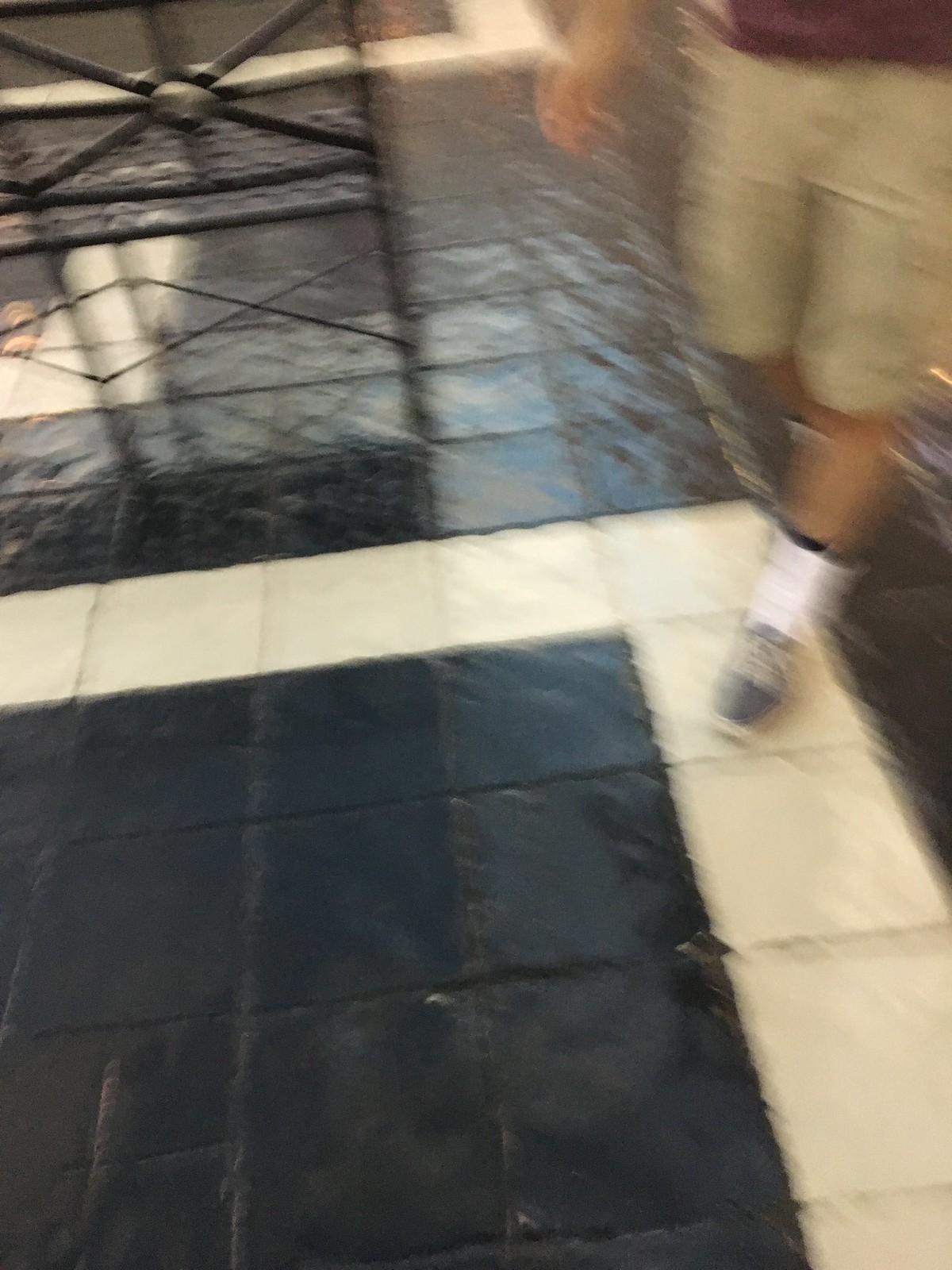This image, slightly blurry but in color, depicts a detailed tile floor that occupies most of the frame. The floor consists predominantly of large, shiny black tiles, accented by a cream-white border forming an inverted L-shape near the center and right side of the photograph. The setting resembles a shopping mall, suggested by a visible metal bench positioned on the tiles and facing an open area.

In the upper right-hand corner, just the lower half of a person is visible. This individual appears to be male and lightly tanned, dressed in white or beige khaki shorts and a maroon or red t-shirt. His attire includes long white tube socks and gray tennis shoes. The photograph is taken straight down at the ground, emphasizing the intricate tile design and the person's casual walk across it. The blurred nature of the image adds a sense of motion to the scene.